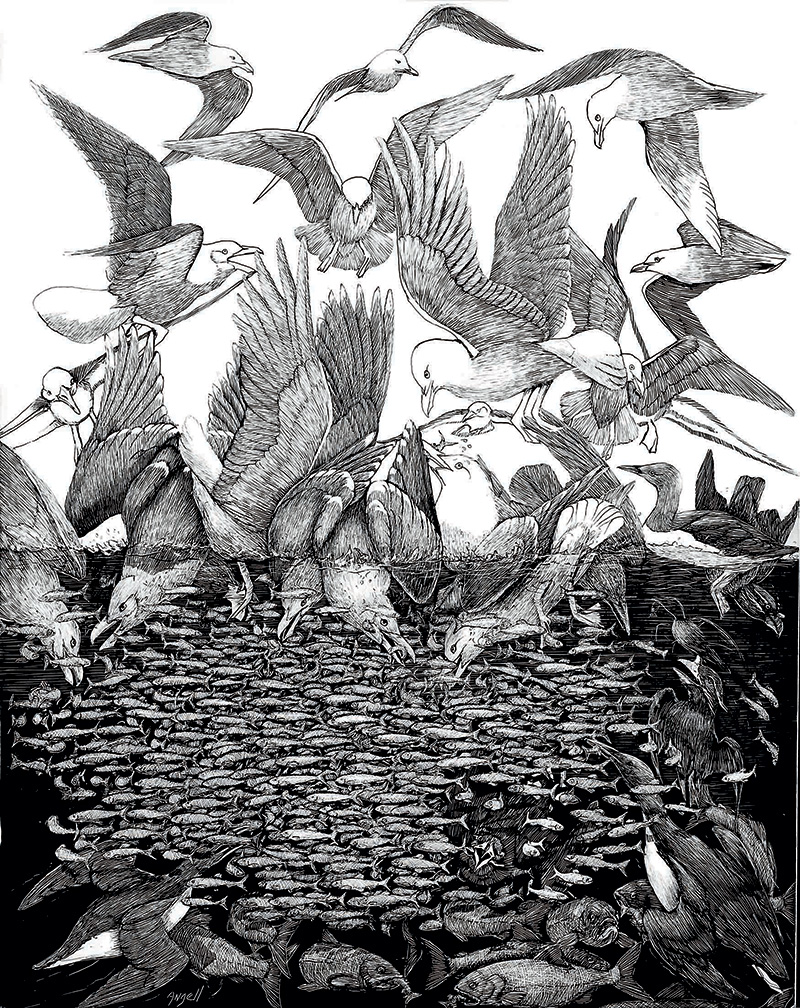The black-and-white image is a detailed, fine ballpoint pen drawing or print capturing a chaotic feeding frenzy of seagulls above and below a body of water. The composition is divided horizontally, with the top half depicting seagulls in mid-flight and diving. These birds, with white heads and gray to black bodies and wings, form an arch in the sky and swoop toward the water surface. Below the water, the scene darkens and becomes more intense as seagulls dive deep, targeting a large circular school of small fish at the center. Surrounding the small fish are larger fish lurking at the deeper depths. The image vividly contrasts the darker underwater scene with the lighter, more dynamic aerial activity above, creating a dramatic visual experience without any text or signature.